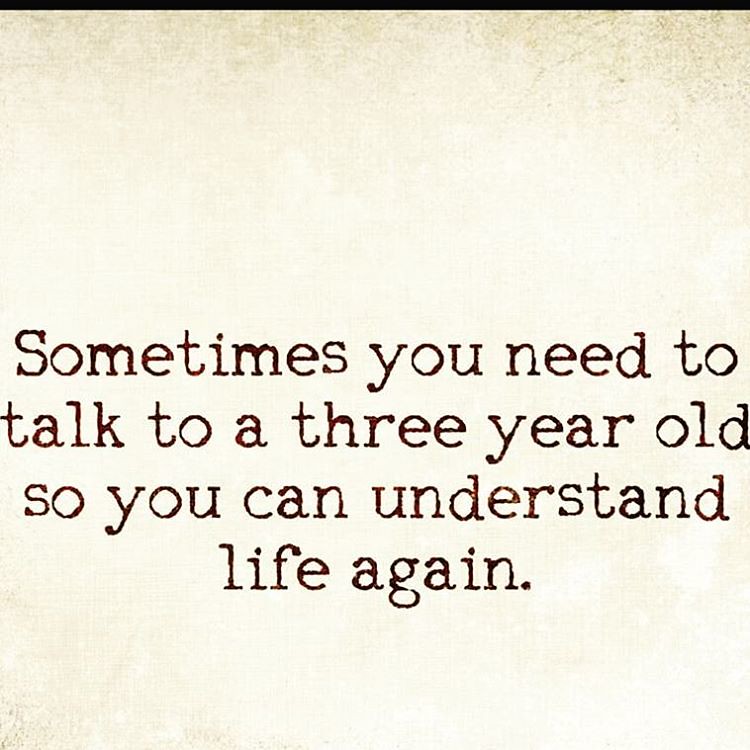This image appears to be a scan of a Facebook post or meme, typically seen as an image macro. It features a motivational quote written in a typewriter-style font, centrally located and slightly more towards the bottom: "Sometimes you need to talk to a three-year-old so you can understand life again." The text is situated over a yellowish-white background that mimics old, aged paper. The background is more worn and damaged near the top, especially where a thin black bar sits at the very top edge of the image. The bottom right corner is the lightest and clearest part of the image, gradually darkening and becoming more distressed as you move upwards. There’s also noticeable JPEG artifacting, indicating image compression. Overall, the image is designed to evoke a nostalgic, old-paper feel, lending a rustic and vintage aesthetic to the digital quote.